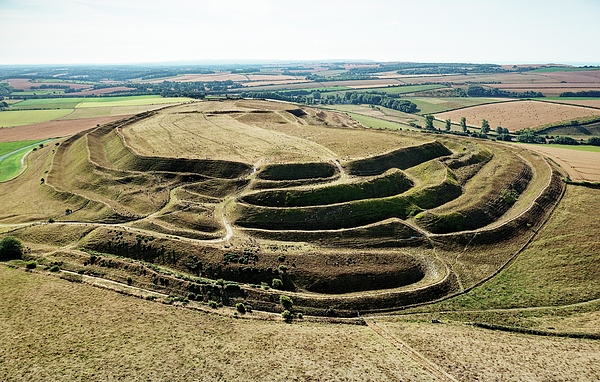Captured in vibrant daylight, this intriguing outdoor photograph depicts an expansive and secluded landscape dominated by farmland. At the center, there is a large, flat-topped mound that stands out prominently against the surrounding scenery. This oval-shaped mound, which could be a historic site, is blanketed in dirt and grass, with smaller mounds cascading down its sides. The mound appears to be intricately layered, with numerous carved roads and creases encircling it, creating a pattern reminiscent of crop circles, though not explicitly defined as such. The image, taken from a considerable distance, reveals compartments and sections within the dirt field, giving the impression of deep divisions. 

Surrounding the mound, vast fields stretch outward, characterized by brown and green patches of grass, interspersed with clusters of lush green trees. The scenic backdrop continues with additional farmland, adding depth to the photograph. The sky above is a serene light blue, dotted with large white clouds, enhancing the tranquility of the rural setting. This detailed landscape, with its layered mound and extensive fields, presents a captivating glimpse into the countryside's natural beauty.